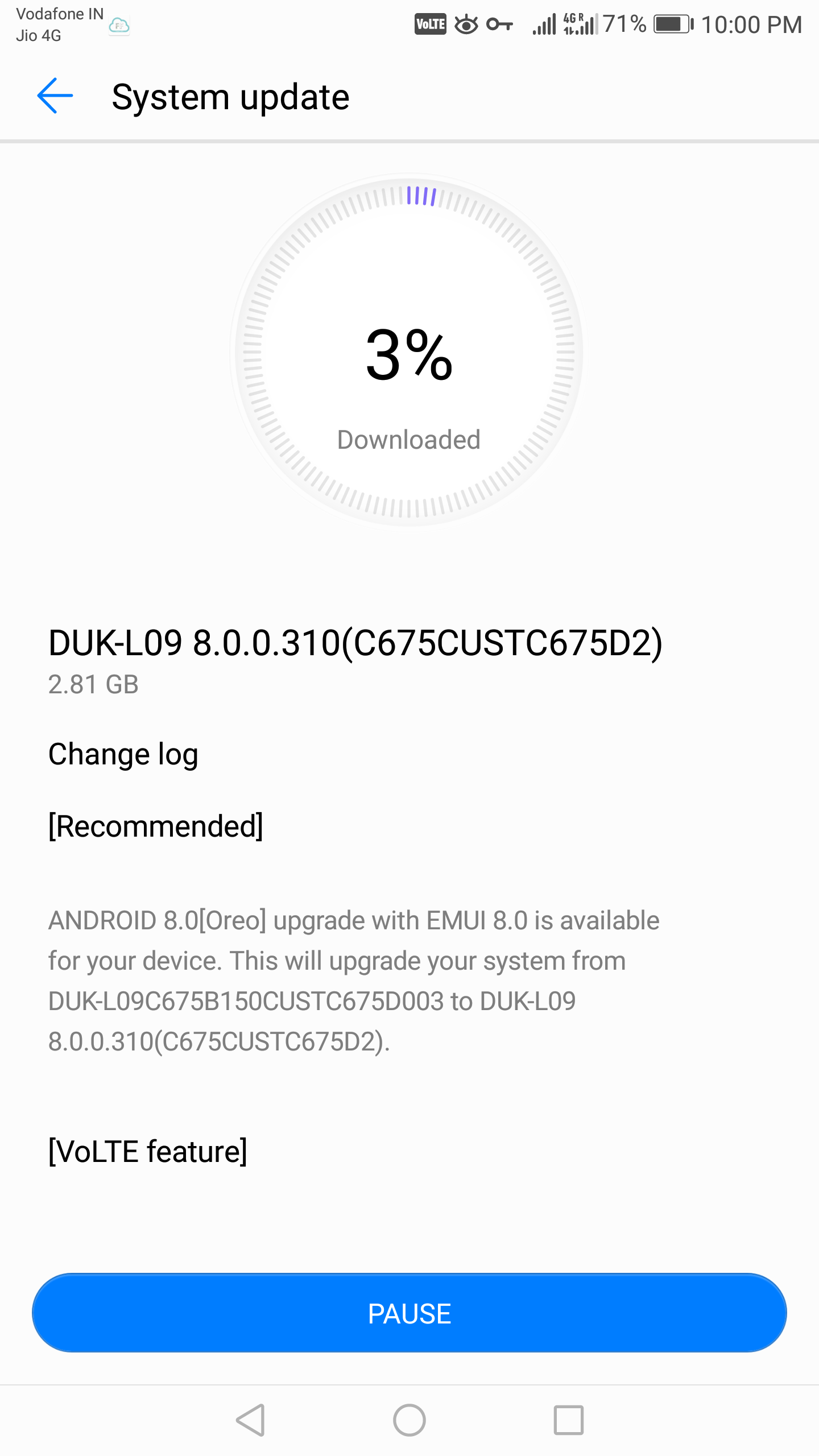The image is a screenshot of a system update page. Located in the upper left-hand corner is a blue back arrow next to the text "System Update." Below this, a circular progress indicator displays the update status, currently at 3% completion, with the percentage figure prominently shown in the center of the circle. Purple progress lines, forming four segments, partially fill the otherwise gray circle to visually represent the download progress. Directly beneath the circle, it states "Downloaded."

Further down, the title and name of the system update are shown, specifying the update size as 2.81 gigabytes. Below this, there is a change log followed by a "Recommended" section that highlights the key feature of the update: an upgrade to Android 8.0 with EMUI 8.0.